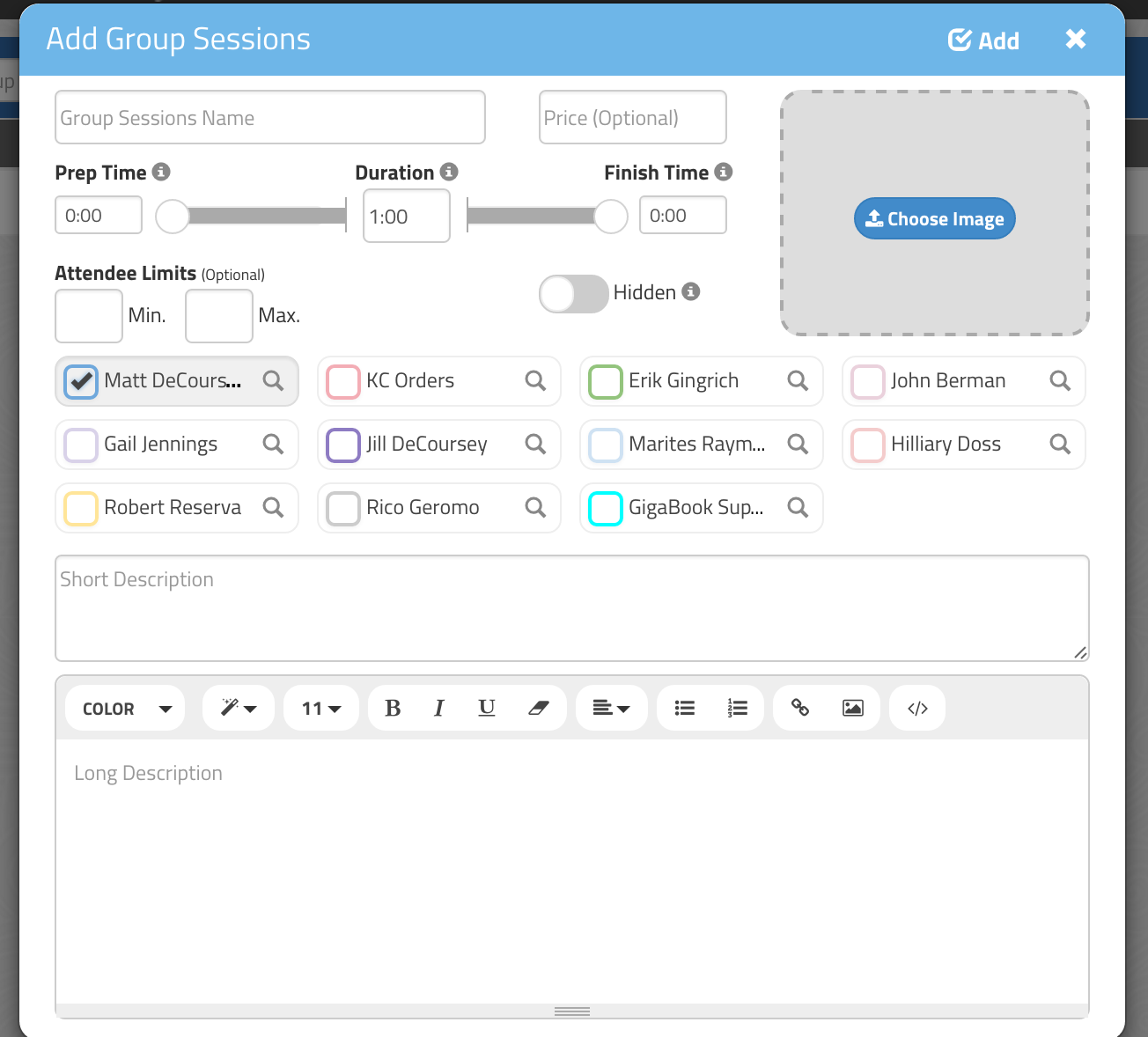This square-shaped photograph captures a user interface screen from an application or web page, focusing primarily on a white pop-up box with a blue header that occupies approximately 95% of the image. The background is grayed out and not clearly visible. The blue header stretches horizontally across the top of the pop-up box, featuring the text "Add Group Sessions" on the left. Adjacent to this text, there's an 'Add' button and a white 'X' button positioned on the right side.

Beneath the blue header, the white background of the pop-up encompasses several interactive elements. At the top, a gray rectangular data entry field prompts the user for "Group Session Name" and an optional "Price." Below this, labeled headers for "Prep Time," "Duration," and "Finish Time" have corresponding editable boxes with sliders for adjusting the values.

Following this section, on the left, a section labeled "Attendees Limits" is visible, which includes input fields for setting minimum and maximum attendee numbers and a toggle switch for "Hidden" that is currently positioned to the left (off). On the upper right of this section, there is a placeholder for an image with a blue rectangular button labeled "Choose Image" in white font.

Further down, the interface displays a list of names highlighted in various colors, likely corresponding to their respective statuses or roles. One name, "Matt DeCourse," is particularly highlighted with a blue box and a check mark inside.

At the bottom, the pop-up features text entry boxes for both a short description and a long description. The long description area includes tools for customizing the font size, color, and text formatting options such as bold, italics, and underline. This detailed interface appears designed for comprehensive session setup and customization within the application.